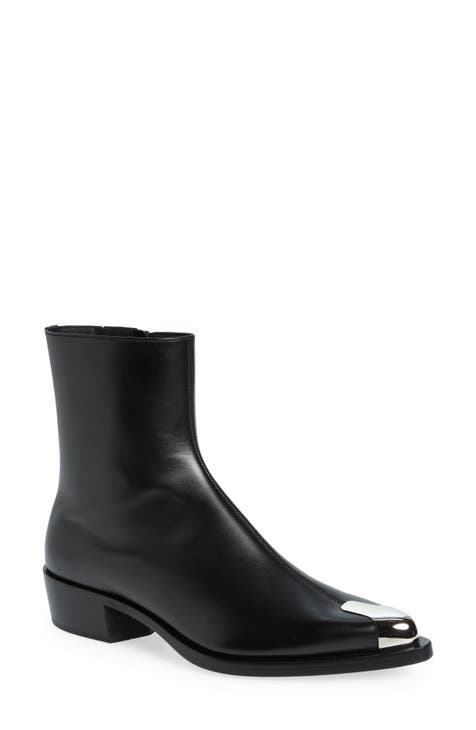This color photograph depicts a single black, ankle-high boot displayed at a slight 45-degree angle against a completely white background. Made from a glossy material, possibly patent leather, the boot features a distinctive black heel approximately two to two and a quarter inches high. The toe area is capped with a notable silver metal piece, extending up along the toe but not too far to the sides. The boot's pointed toe and sleek design suggest a unisex style, and it appears to zip up on the far side from the viewer, indicating it is a right boot. The heel and sole are distinctly separate from the upper part of the boot, adding to its structured appearance. Some light reflection off the glossy surface and the metal cap enhances the boot's sharp and polished look.